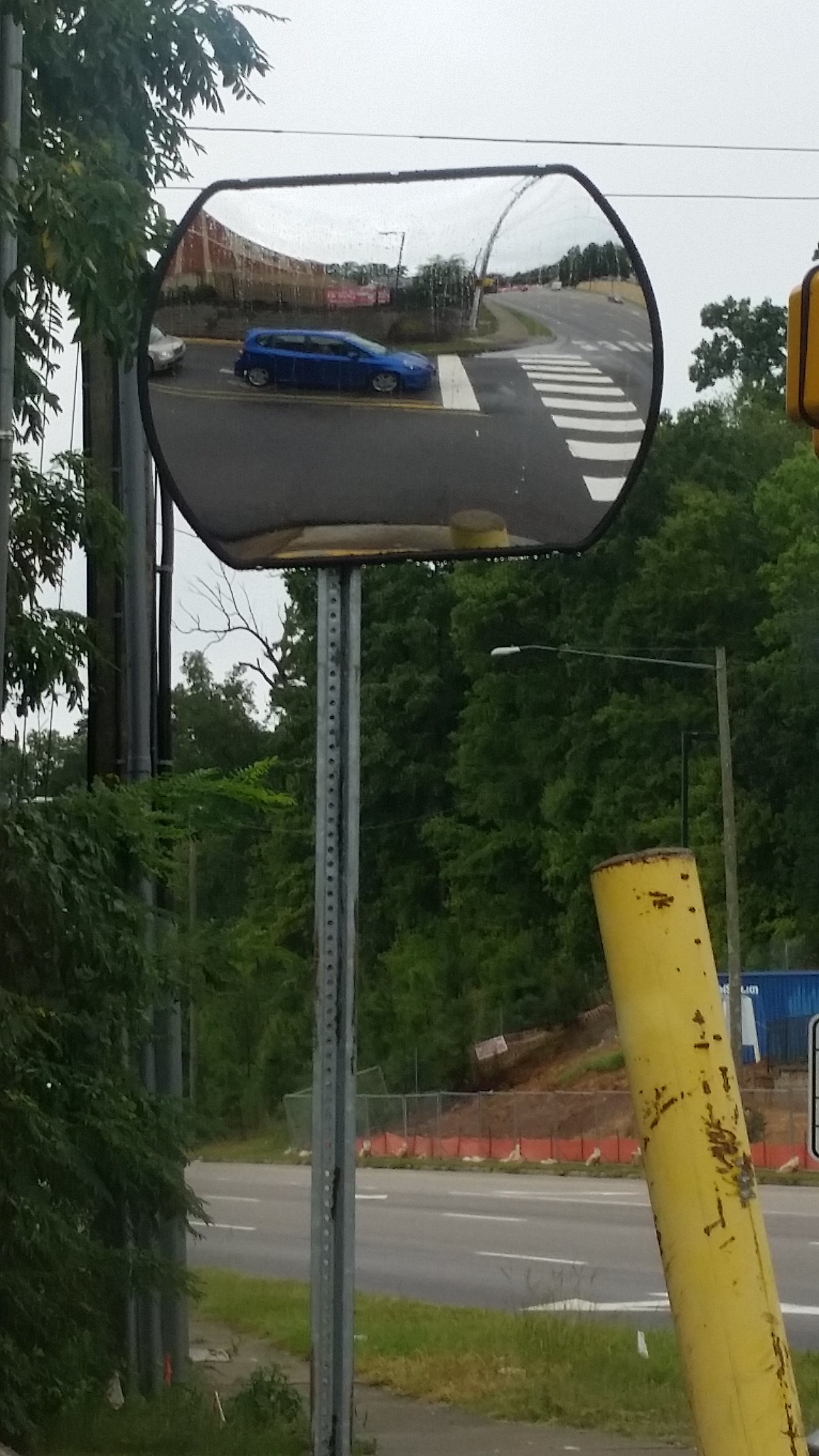This photo, taken outdoors on an overcast day, captures a street corner scene with a large, rectangular mirror mounted on a silver metal post to assist with visibility at a blind intersection. The mirror, which has rounded ends, reflects a blue four-door hatchback at a white crosswalk marked with dashed lines, along with a silver car and part of the street. In the foreground, to the right, a large, yellow, dinged-up metal pole emerges from a grassy and dirt-covered ground at a slight angle. The mid-ground features a gray asphalt road with white lane markers crossing the image. On the left-hand side stands a power pole, while the scene includes tall trees with bright green leaves and a light gray sky above. Across the street, a fenced-off construction area is visible, with orange plastic fencing at the bottom and a blue metal garbage can within. In the background, the mirror also reflects additional elements, including a brown building and a continuation of the street.